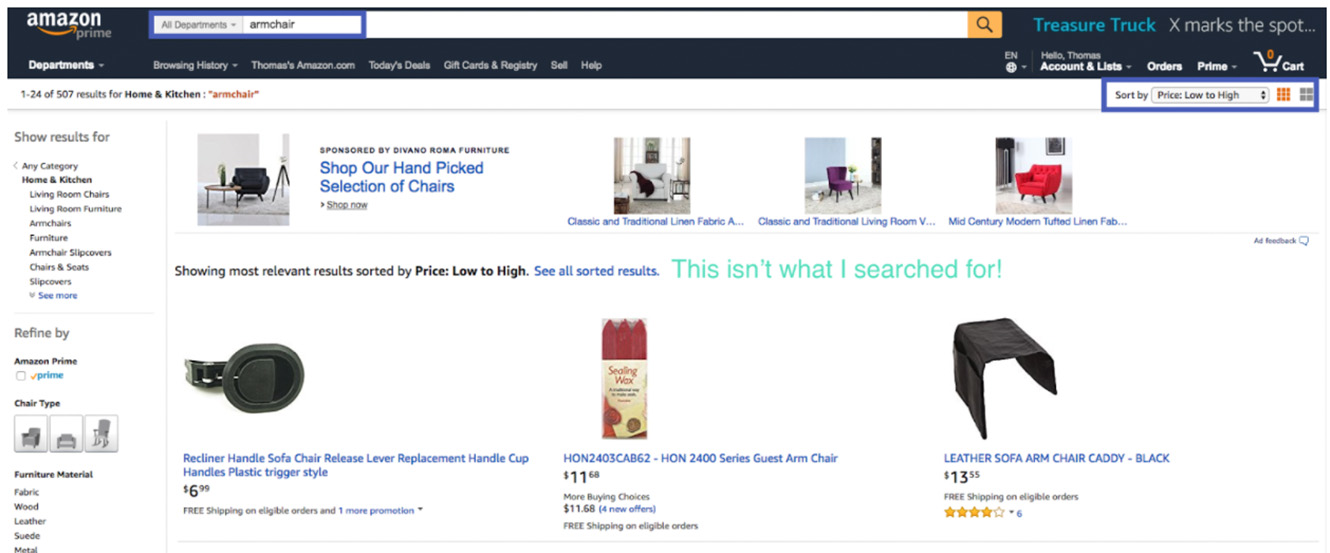Sure, here is the cleaned-up and detailed caption:

---

This image shows an Amazon webpage where a user has searched for "armchair" under the "All Departments" category. The top area of the screen is black, featuring the Amazon logo and navigation options such as "Account & Lists," "Orders," and "Cart," which indicates zero items. The search bar, located at the top center, is white with a yellow square at its right end containing a magnifying glass icon. 

In the search results, various products related to armchairs are displayed. One item is a recliner release lever replacement handle available at $6.99. Another product is a series guest armchair wax priced at $11.68. Additionally, there is a black leather sofa armchair caddy listed for $13.55. 

The webpage also highlights other functional features, including a section where a rectangle has been drawn around the sorting option "Sort by: Price: Low to High." The page greets the viewer with "Hello, Thomas," indicating the logged-in account, and shows sections for Prime memberships and other account-related options.

---